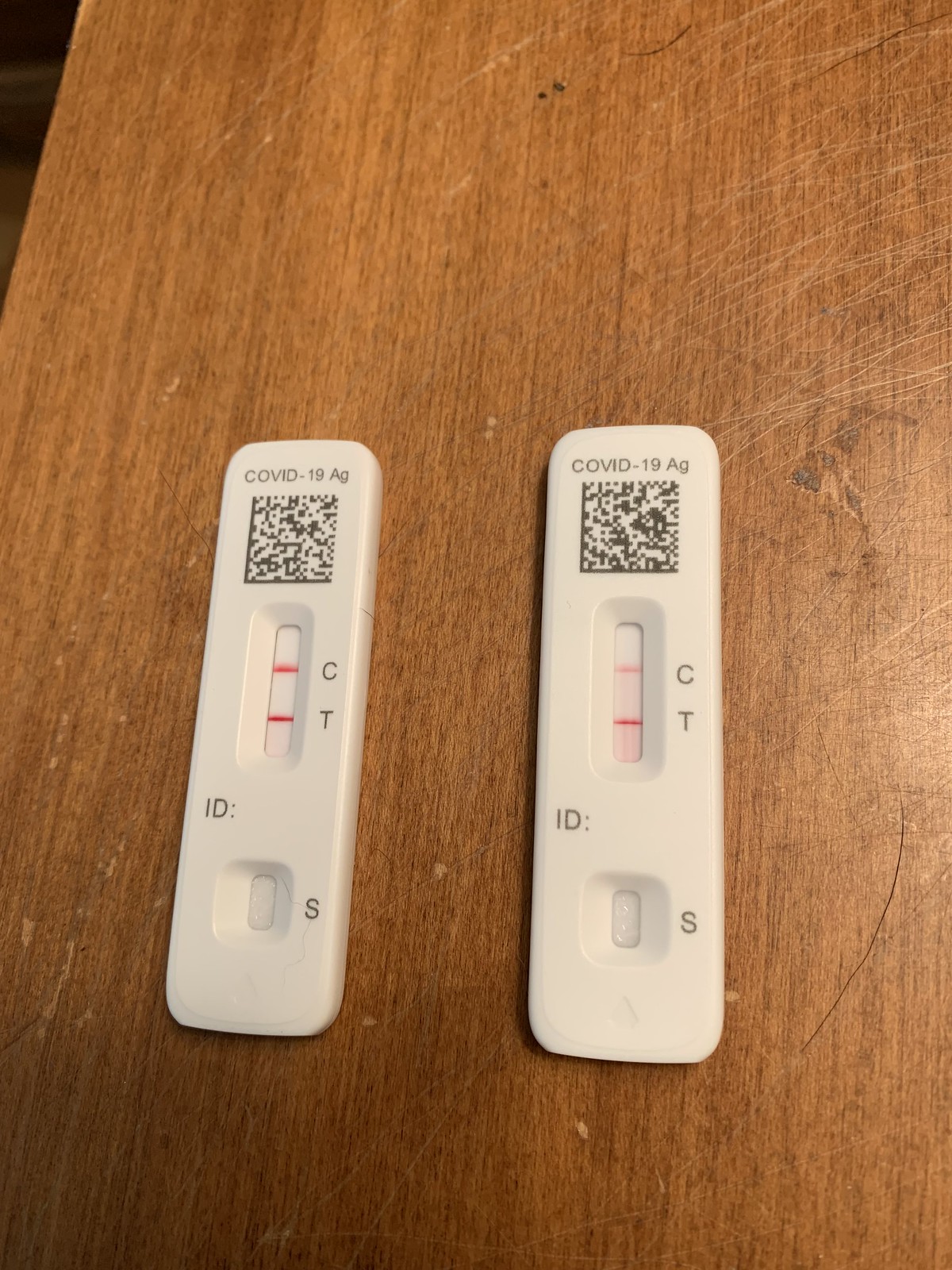The photograph features two rectangular COVID-19 test kits laid out on a weathered, scratched wooden surface. Each test kit is predominantly white with black markings, and prominently labeled "COVID-19 AG" at the top. Adjacent to the label, there is a QR code designed to direct users to a specific webpage when scanned. 

Below the QR code, each test has a results window displaying two red lines. The upper line, labeled "C" for control, indicates the test's functionality, while the lower line, labeled "T" for test, reveals the test outcome. Both kits exhibit two red lines, signifying positive test results for the presence of the virus.

Further markings include the letters "I.D." situated below the results window, and another, empty window labeled "S" at the bottom. Notably, the test on the right features a fainter "C" line and a pink-tinted background within the results window, contrasting with the plain white background and sharper red lines of the left test.